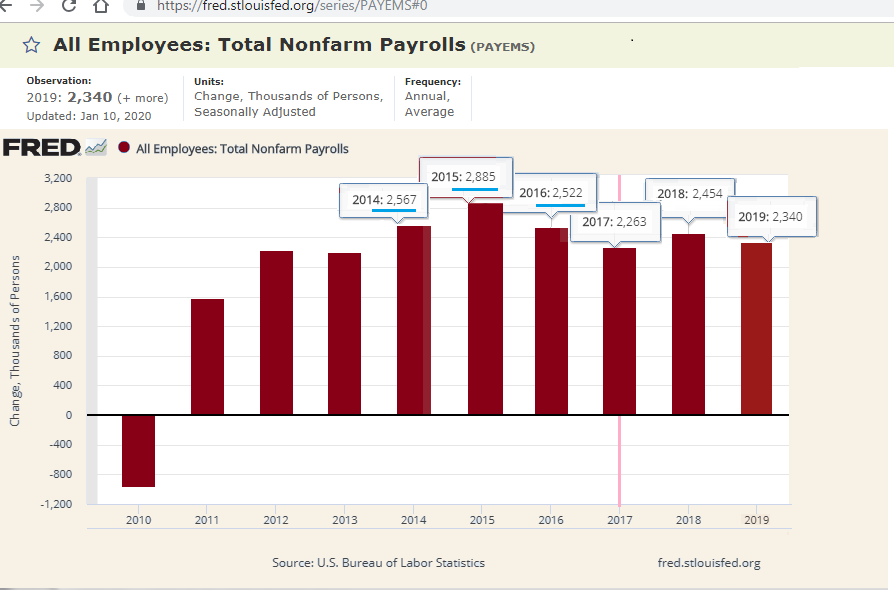The image is a screenshot captured from a computer screen, depicting a detailed chart from the website fred.stlouisfed.org. The chart, titled "All Employees: Total Non-Farm Payrolls," includes various metrics such as observation units, frequency, and annual averages, with data spanning from 2010 to 2019. The chart is centrally positioned on a white background, with navigation elements like the back or refresh button visible at the top, indicating it was taken from a website. The source is cited as the US Bureau of Labor Statistics.

The chart features a bar graph illustrating changes in thousands of employees, ranging from -1200 to 3200. Years are marked along the bottom, with significant observations noted: a low in 2010, a rise through to 2014, a drop in 2016, followed by fluctuations in the following years. Red measurement lines run vertically across the screen to aid in data comparison. The colors present in the image include gray, black, green, white, red, light blue, and tan, contributing to the chart's readability.